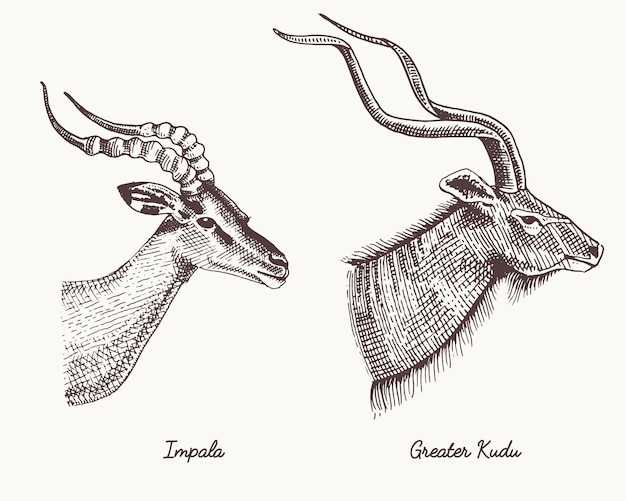The image features detailed black and white sketches of two distinct deer-like animals, set against a tan background. The left side of the image is labeled "Impala," showcasing a sketch of an animal that resembles a deer, characterized by cross-hatched shading and unique, bubbly horns that appear as if marshmallows are stacked along their length. The Impala also has pointy ears. On the right side, the label "Greater Kudu" identifies a sketched head of an animal that looks like a cross between a goat and a horse. This creature is depicted with long chin hairs extending down its neck, and it boasts significantly longer, spiraling horns compared to the Impala. The Greater Kudu's ears are noticeably less pointy.